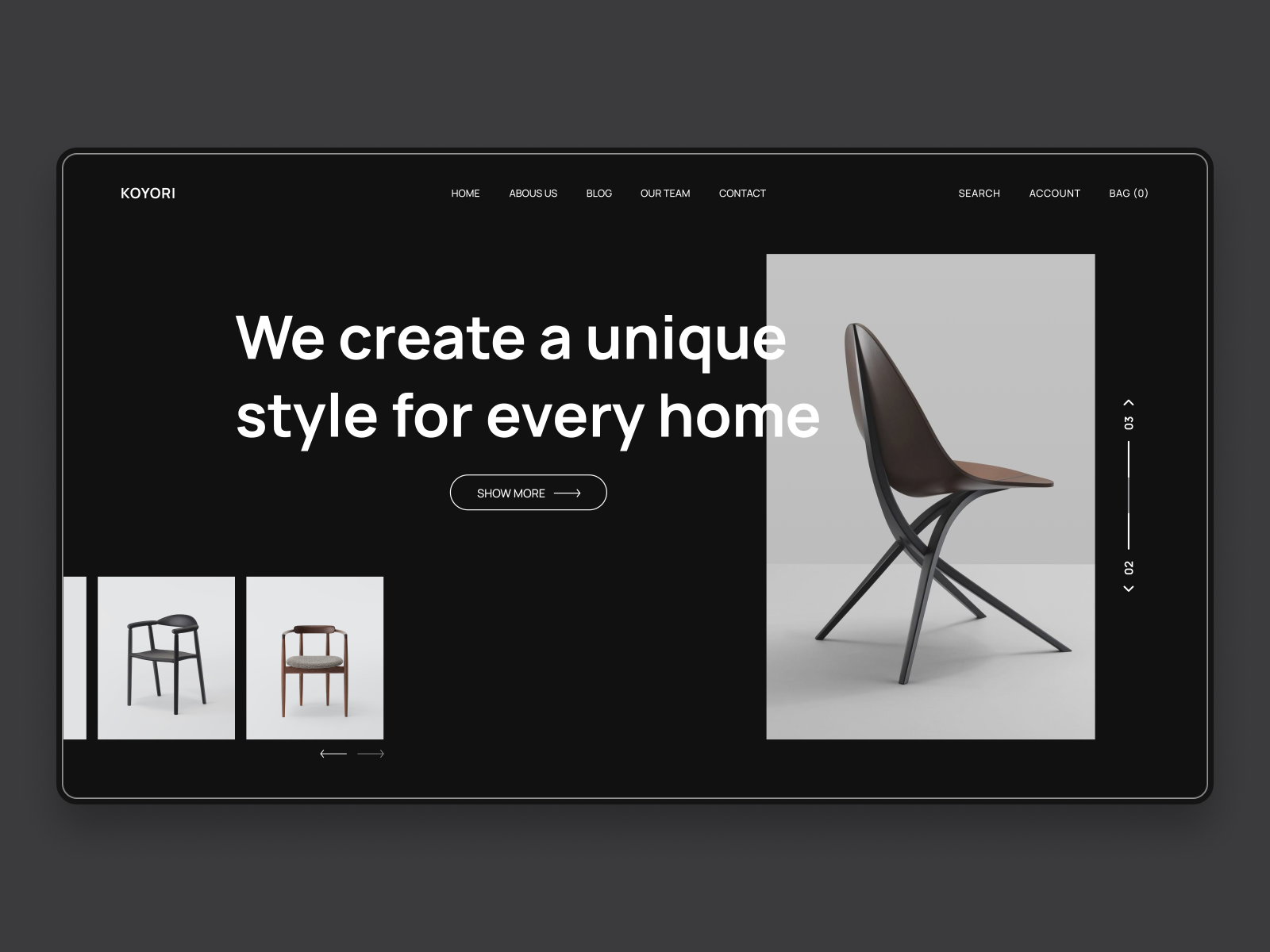An advertisement displayed on a dark gray background, featuring the image of a tablet laying flat. The left side of the tablet shows a jet-black background, while the right side combines jet-black edges with a gray-outlined image. 

Across the top of the tablet screen is the brand name "Coyori" in white lettering. Below this, a menu bar lists "Home," "About Us," "Blog," "Our Team," and "Contact," all in white. Further to the right, icons for "Search," "Account," "Bag," and "(0)" are also displayed in white.

The center of the screen features a bold white text reading, "We create a unique style for every home." Directly beneath this statement is an oval button labeled "Show More" in white, with an arrow pointing to the right.

In the bottom left corner of the image are two smaller images featuring chairs that resemble stools but are the height of regular chairs, set against a white background. Dominating the far right side of the screen is a large, gray-outlined image of a highly modern, walnut wood chair with a high-tech appearance. The chair's sleek design is highlighted by its placement amidst four interweaving pieces of gray steel.

On the right side of the tablet screen, a white arrow points downwards with a corresponding upward white arrow. A white line connects these arrows running vertically, indicating navigation through different sections. The bottom of the line is marked "02" and the top "03".